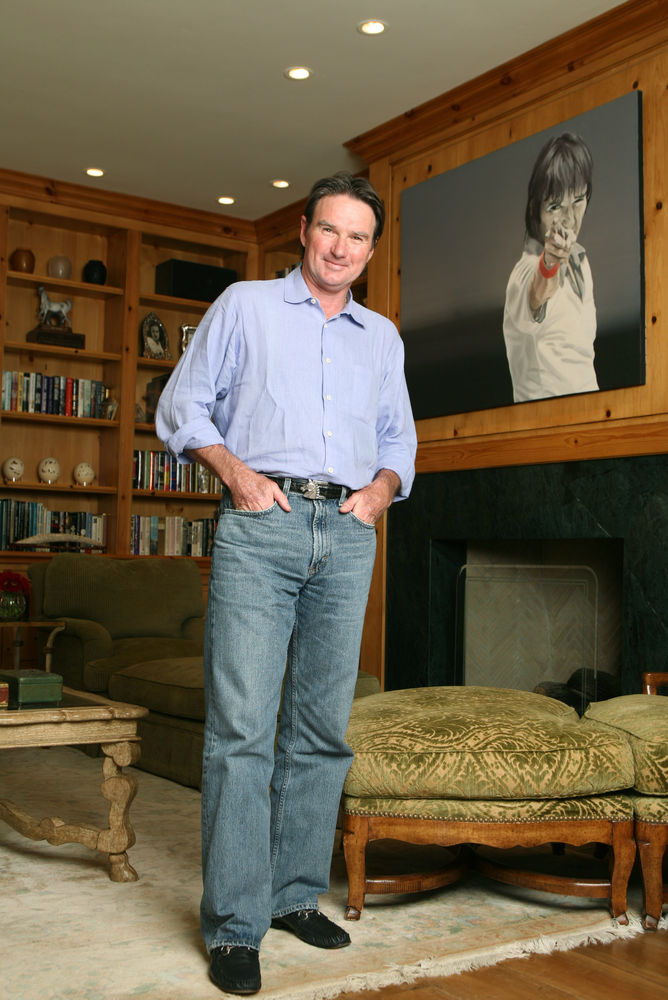The photograph captures a clean-shaven man with short dark hair standing in the center of a well-furnished, warmly lit room. He is smiling at the camera, wearing a light blue button-down shirt with the sleeves rolled up to his forearms, blue jeans, a black belt, and black shoes. His hands are tucked casually into his pockets. The room features rich wood paneling, a comfortable warm ambiance, and several pieces of furniture, including a coffee table, stools, and a brown sofa. Behind the man is a bookshelf lined with books and various items, and to his right, a painting or photograph of another man with black hair and a white shirt, who is pointing. Adjacent to this painting is a fireplace, above which hangs the artwork. Adding to the cozy decor is a large, plush beige carpet that covers the wooden floor. The ceiling has lights that softly illuminate the space, blending seamlessly with the overall inviting theme of the room.